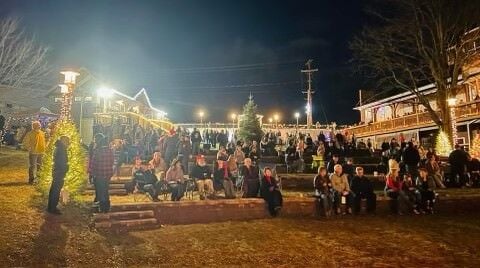This nighttime photograph captures a bustling hometown gathering in the heart of a town, possibly a festive Christmas event like a tree lighting ceremony. The scene is illuminated by numerous bright lights adorning various buildings, which might be businesses. A large crowd, likely over a hundred people, is seated on sidewalks, brick ledges, and chairs, with a few standing and engaging in conversation. The attendees are bundled up in winter attire, featuring a rainbow of colorful jackets—reds, whites, blacks—and a mix of pants including black, blue jeans, denim, white, gray, and khaki. Notably, some men sport red flannels, and a gentleman on the far left wears a distinctive yellow sweatshirt. Bare trees and a few Douglas firs, although not decorated, are visible among the power poles and buildings. A prominent three-story structure on the right has people on its balconies, all basking in the luminous setting. The dark sky underscores the cold, wintry night, yet the vibrant lights envelop the scene in a warm, festive ambiance.